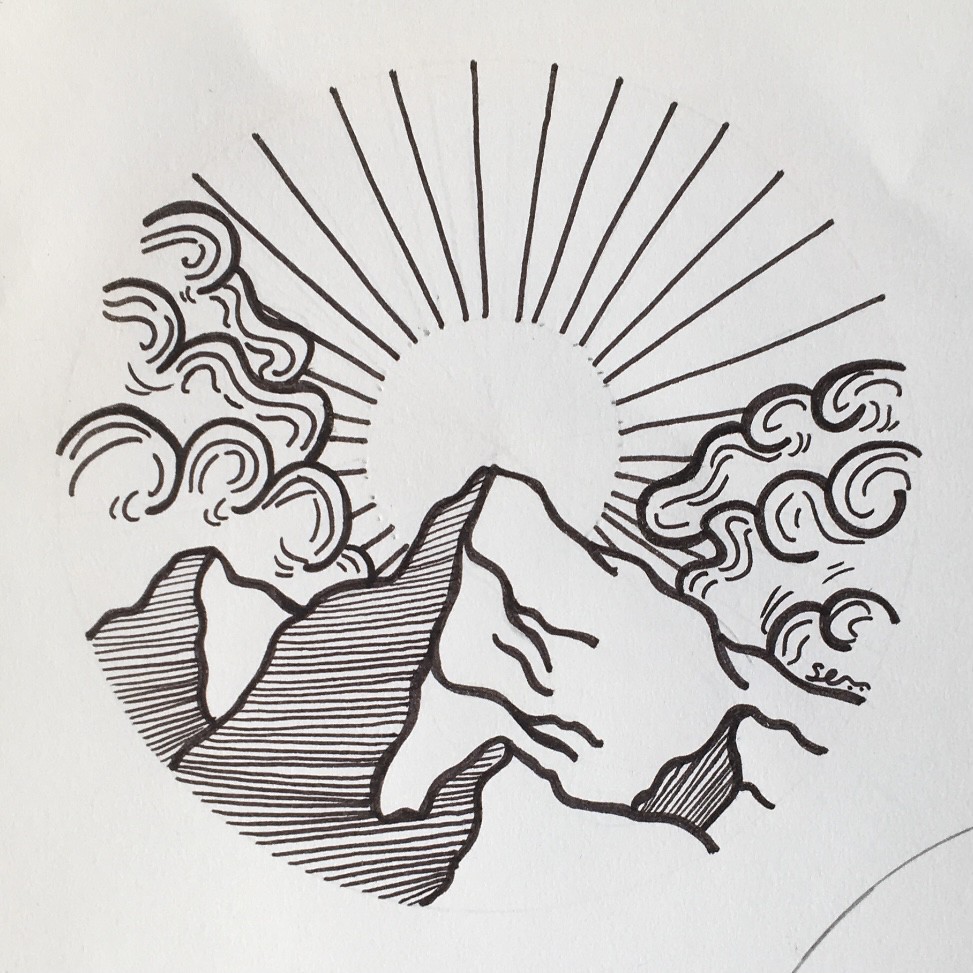This artwork appears to be either a detailed coloring page or an individual's black marker drawing. At the center of the composition is a large depiction of the Sun. The artist has left the middle section of the Sun white, circumscribed by an array of black marker lines that radiate outward, symbolizing sunbeams. On either side of this radiant Sun, large, wispy, curly formations suggest the presence of clouds, adding depth and movement to the piece.

The lower portion of the drawing features a range of mountains, partially obscuring the Sun and nestled between the clouds. The mountains are rendered with notable attention to shadowing; the left side of the largest mountain, and similarly the smaller mountains to its right, are accented with black stripes to create the illusion of shadow.

Finally, while the image lacks a traditional border, the edges of the drawing come together in such a way that it subtly forms a circular frame around the entire composition. The meticulous detailing and stylistic touches in the artwork create a visually striking and cohesive scene.